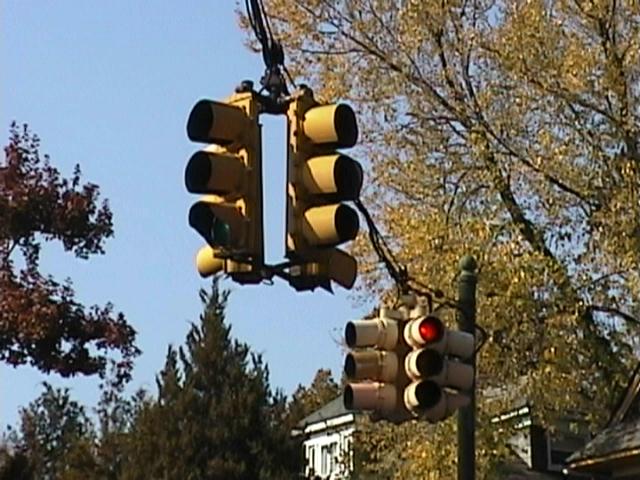This color photo depicts an outdoor autumn scene in a town, showcasing two traffic lights suspended from a cable stretched across the street. Both traffic lights hang loosely from the cable attached to a visible dark pole, with one light clearly showing red, while the other is angled such that its signals are not visible. The scene is set under a clear, vibrant blue sky without any clouds, and includes a mix of trees; to the left, coniferous pines display their evergreen needles, while a tree with reddish leaves and another to the right with extensive yellow foliage add to the seasonal ambiance. In the background, there are several houses, including a white one partially obscured by branches. The lower resolution of the image slightly blurs the details, but you can distinguish that it's a four-way intersection. The bottom right corner of the image also reveals a glimpse of shingles, likely from another nearby home or building.